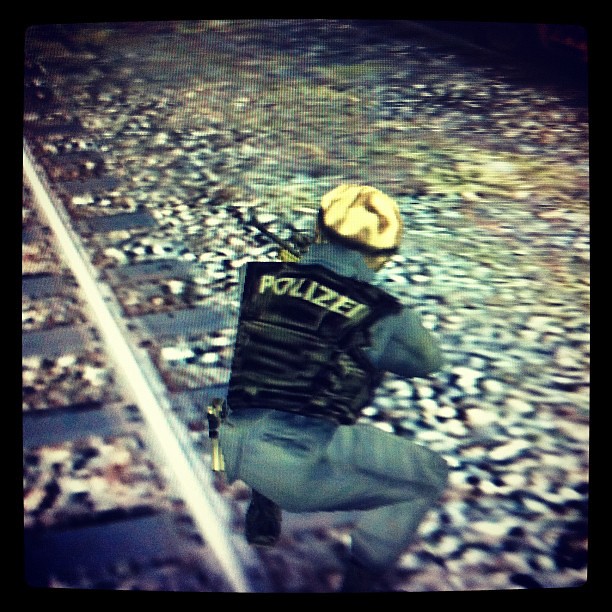In this pixelated image, the central focus is on a person dressed in a police uniform. The individual, identified by the "Polizei" label on their black vest, is crouching near a visible section of a railroad track, which features one of the rails and several crossboards on the left side of the frame. The person is dressed in a yellow or gold cap, a light blue shirt, and blue pants, along with black shoes. The background on the right side displays a textured stone surface, enriched with a blend of colors, including purple, yellow, turquoise blue, and white. The image is notably pixelated, signaling it is likely not a high-resolution photograph.